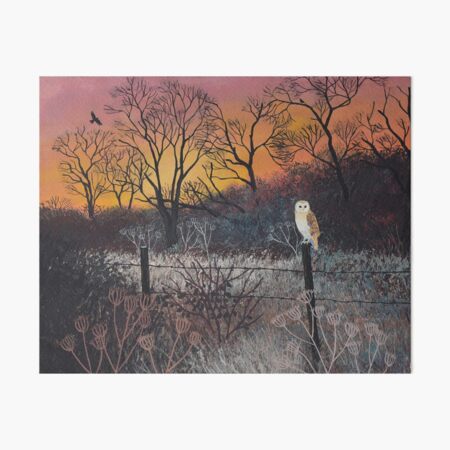In this hand-painted image, an owl perches majestically on a weathered wooden fence post, the post part of a barbed wire fence that stretches through a meadow-like landscape. The owl, with its striking white stomach and light brown feathers, has piercing black eyes that gaze out into the distance, possibly scouting for its evening meal. The surroundings are wild and untamed, with a mess of reeds and bushes flanking the fence, and the ground dotted with shrubs and whippoorwills.

The setting appears to be late fall or winter as the towering trees in the background stand bare, their branches a stark blackish-brown, devoid of any leaves. These leafless sentinels rise from a small hill that slopes gently from the left to the right of the scene, adding to the serene, almost melancholic atmosphere. The sky is a breathtaking gradient, transitioning from a pale pink at the top to a rich orange near the horizon, suggesting a beautiful sunset. Far in the distance, smaller birds, possibly hawks or crows, are seen flying, adding a sense of depth and movement to the tranquil evening scene.